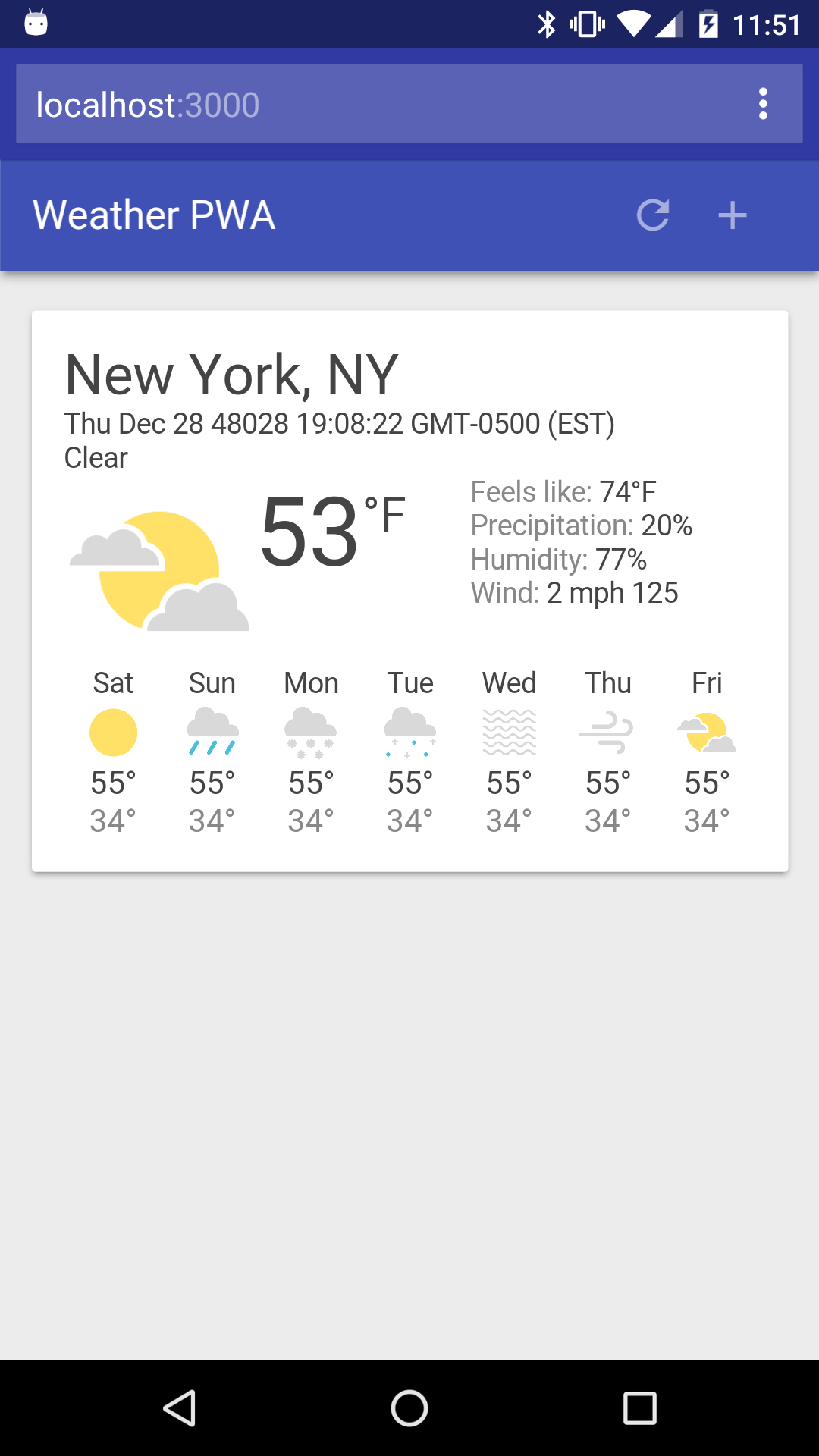The image is a screenshot of a weather website, captured on a cell phone, evidenced by its long and narrow dimensions. At the top of the screen, a small, robot-like icon is visible, accompanied by various status indicators on the right side such as a Wi-Fi symbol, signal bars, battery level, and the time, which reads 11:51. The website's URL is displayed as "localhost:3000". On the right side of the header, there is a "More" button denoted by three vertical dots.

Below the header, the app title "Weather PWA" appears, alongside a refresh icon (a circle with an arrow) and a plus sign. The main section of the screenshot presents the current weather for New York, New York on Thursday, December 28th. The zip code is listed as 48028, and the time is presented as 19:08:22 GMT-0500 Eastern Standard Time (EST). The weather condition is described as clear, with an accompanying icon of a sun partially obscured by clouds. The temperature is noted as 53°F, feeling like 74°F. Additional weather details include a 20% chance of precipitation, 77% humidity, and wind speed at 2 mph from a direction of 125°.

The image also includes a weekly forecast:
- **Saturday:** Sunny with a high of 55°F and a low of 34°F, represented by a sun icon.
- **Sunday:** Cloudy with rain, high of 55°F and low of 34°F.
- **Monday:** Cloudy with potential snow, indicated by little gray drops, high of 55°F and low of 34°F.
- **Tuesday:** Mixed rain and snow, shown by gray and blue dots, high of 55°F and low of 34°F.
- **Wednesday:** Possibly windy, suggested by squiggly lines, high of 55°F and low of 34°F.
- **Thursday:** Stronger wind, conveyed with larger wavy lines, high of 55°F and low of 34°F.
- **Friday:** Partly cloudy, high of 55°F and low of 34°F.

The consistent high and low temperature of 55°F and 34°F across the week raises some suspicion. At the bottom of the image, there is a black navigation bar featuring a left arrow, a circle, and a square.